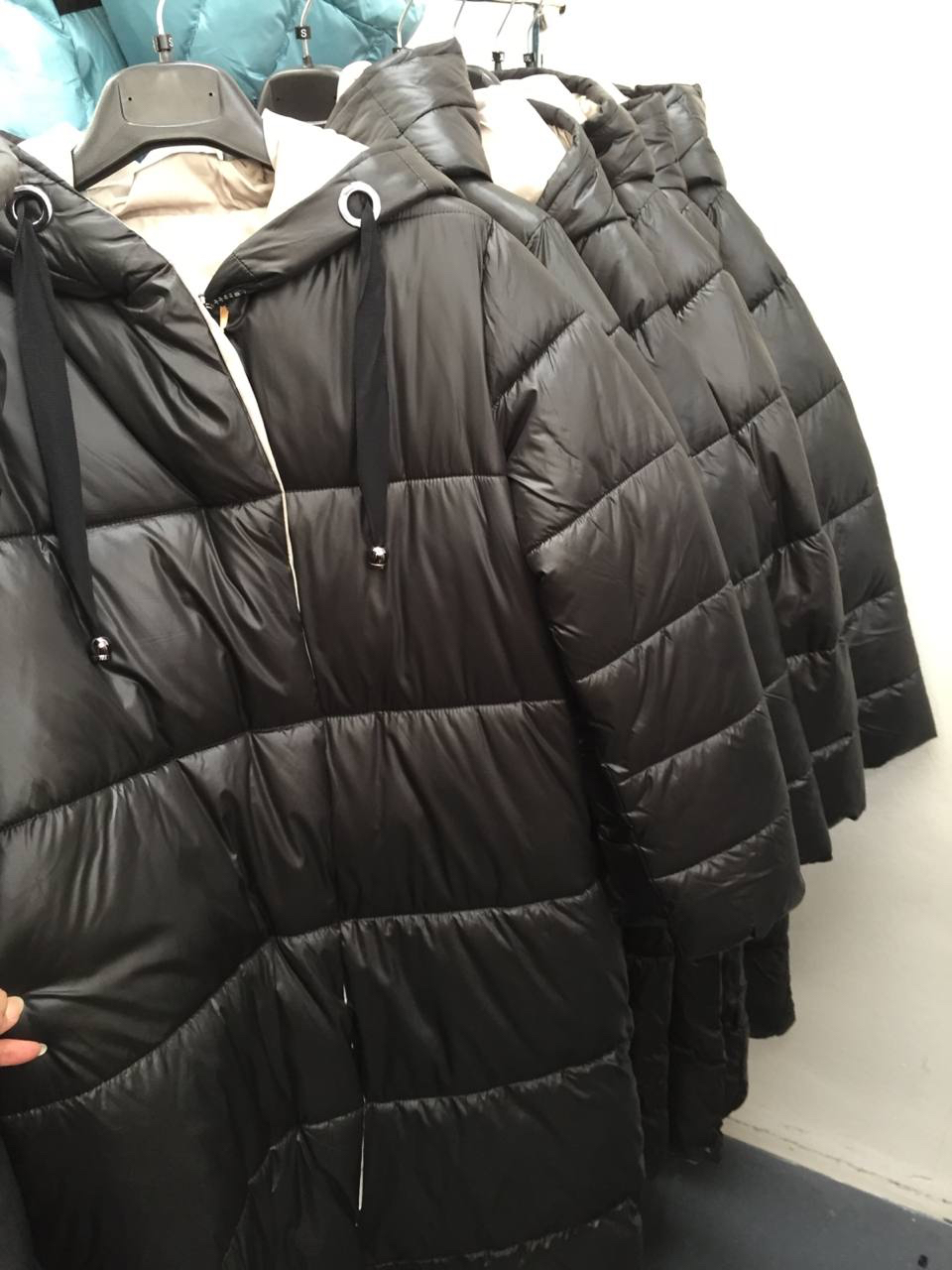The image depicts a group of approximately half a dozen identical black puffer-style jackets, each featuring horizontal quilting lines around the torso and sleeves. The hooded jackets have black laces with silver aglets threaded through silver grommets at the base of the hoods and are lined with a light-colored fabric. They are all hung on black plastic hangers with metal hooks. A light-colored wall and a dark-colored floor are visible on the right-hand side of the image. At the top, part of a similar jacket in an aqua color is seen, while at the lower left-hand edge, a few fair-skinned fingers with long fingernails point to one of the jackets. This image appears to be taken indoors, possibly in a shop, given the arrangement and display of the jackets.